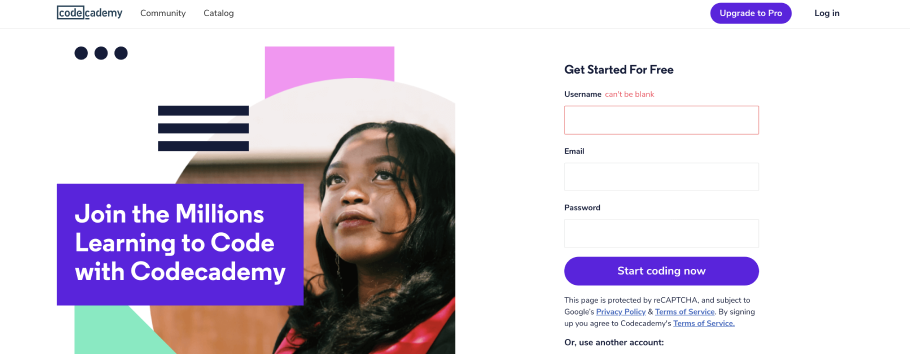The image displays a Codecademy webpage with a clean, white background. In the top left corner, the Codecademy logo is prominently featured in dark blue, encapsulated within a blue square. To the right of the logo are two navigation tabs labeled "Community" and "Catalog."

On the top right, a prominent purple button with white text invites users to "Upgrade to Pro." Directly to the left of this button is a black "Login" button. Dominating the right side of the image is the sign-in section, headlined with "Get Started For Free." 

A username field is outlined in red, accompanied by the error message "Username can't be blank" in red text. Below this field are additional input areas for "Email" and "Password." Towards the bottom of the sign-in section, a green button encourages users to "Start Coding Now."

The page also mentions that it is protected by reCAPTCHA and includes annotations about Google’s Privacy Policy and Terms of Service. Text at the bottom states that by signing up, users agree to Codecademy's Terms of Service and are given the option to use another account.

On the left side of the image, against a purple background, white text reads: "Join the millions learning to code with Codecademy." Below this informative text, there is an image of a student dressed in black and red, with long black hair, visually reinforcing the call to join the coding community.